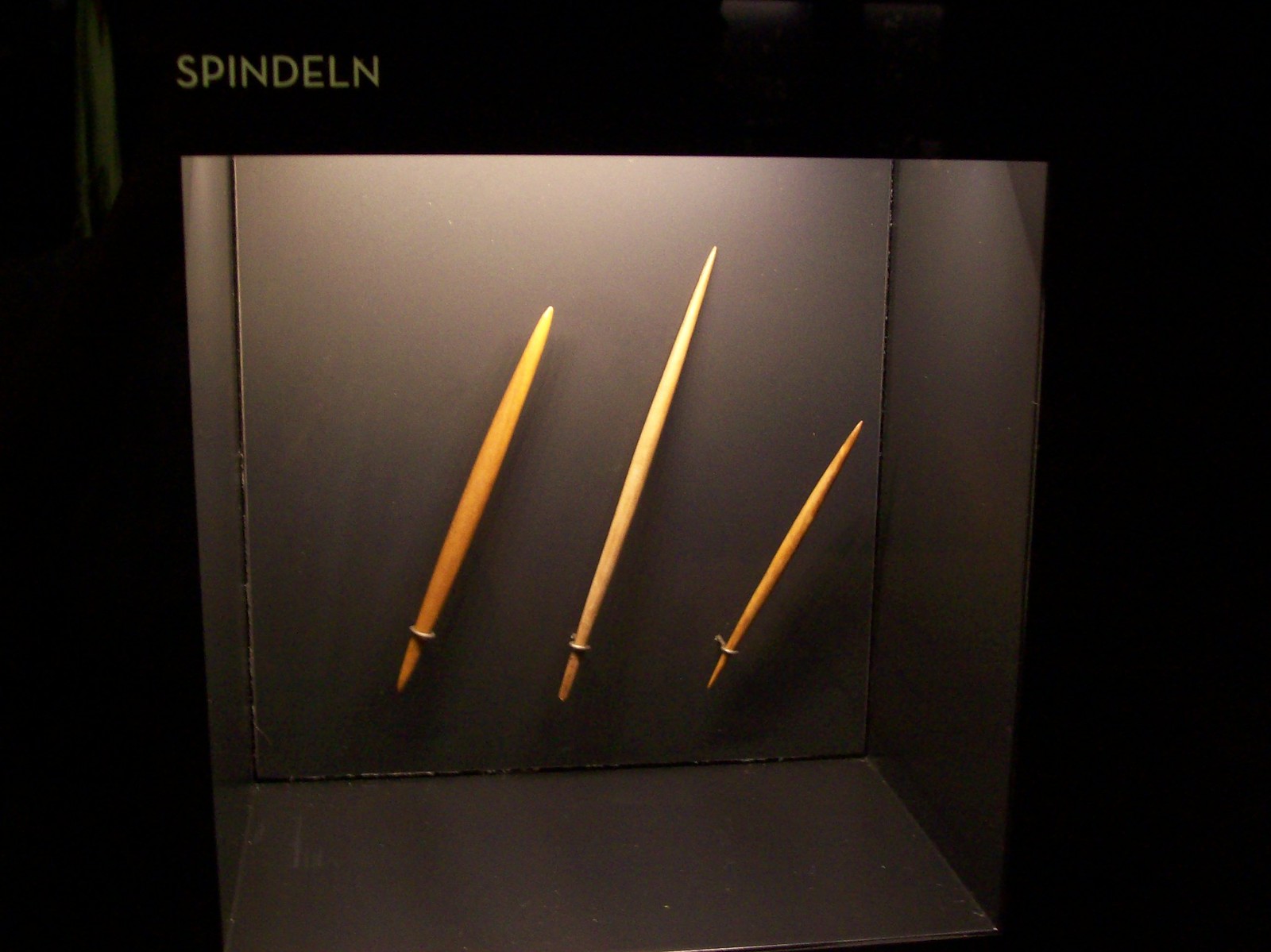The image depicts a black display box with open front and top, possibly showcased in an art exhibition. Inside this well-lit box, there are three wooden sword-like objects, mounted at a rightward slant by small metal holders attached to the back wall. Each object has pointed tips and varies in size and color. The leftmost is golden-yellow and of medium length, the center one is tan and the longest, and the rightmost is the smallest, also featuring a golden-yellow hue. The background of the box is dark black, which contrasts with the three objects. At the top left corner, the word "SPINDELN" is prominently displayed in all caps with a yellow mustard hue. The bottom of the box reveals dark gray flooring and matching dark gray walls, illuminated by white light from above, highlighting the contents effectively.